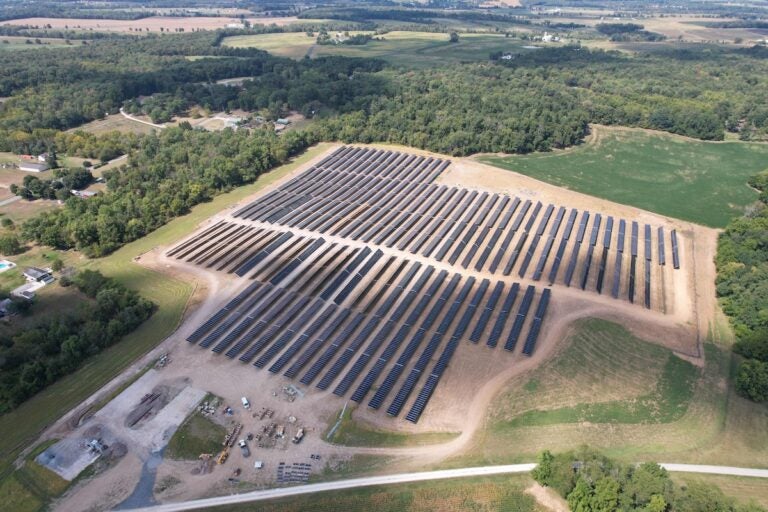This is an aerial view of a solar farm situated near a large forest. The background of the image features dense trees and foliage, interspersed with smaller buildings or houses tucked amongst the woods. Off to the left, additional smaller structures are visible. The bottom of the image showcases a curved road that transitions into a wider paved road, leading into the main area of the solar farm. The farm comprises approximately nine rows of solar panels, with each row arranged meticulously to maximize sunlight collection. The first and fifth rows are of similar shorter lengths, while the second through fourth rows are the longest. The solar panels, black and angled towards the sky, are divided between areas of sunlight and shade due to clouds rolling through on this sunny day. This multi-million dollar facility is capable of producing significant amounts of electricity, leveraging the solar energy collected by these numerous rows of solar strips.